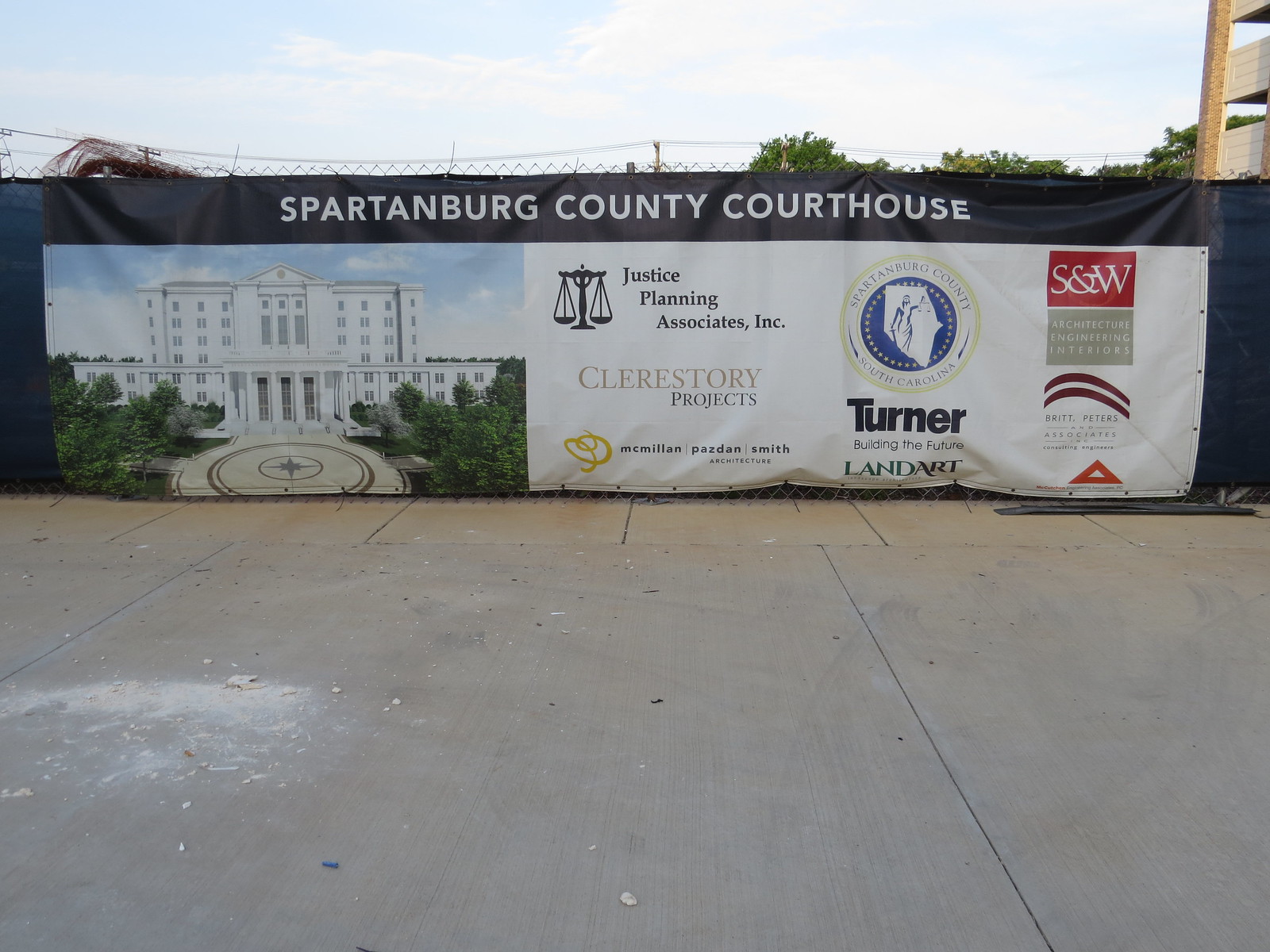The photograph captures a vibrant outdoor scene at a construction site. Most of the image is dominated by a long, large vinyl banner attached to a fence, which encloses the construction area. Above the fence, light blue skies with sparse, fluffy clouds and tree tops peek through. The focal point of the banner is a black section at the top, featuring the bold white text "Spartanburg County Courthouse." Below this, on the left side of the banner, is a detailed digital rendering of the future courthouse building. The rendering depicts an imposing white structure with seven stories, a grand pillared entrance, and a spacious round walkway flanked by trees, suggesting a sense of grandeur and civic pride.

To the right of the image on the banner, a white background lists the sponsors and firms involved in the project, including Justice Planning Associates, Inc., Clarestory Projects, McMillan-Pazdan-Smith Architecture, Spartanburg County, South Carolina, with their logo, Turner, Building the Future, Land Art, S&W Architecture Engineering Interiors, and Britt Peters Associates. The banner is secured to the fence with visible grommets, giving a professional and orderly appearance. The lower part of the photograph shows the cement sidewalk, emphasizing the integration of this future courthouse within the existing urban landscape.